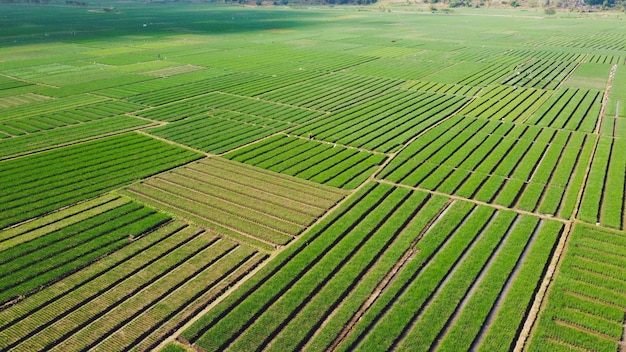This aerial shot captures an expansive farmland with neatly organized rows of diverse plants. The farmland stretches as far as the eye can see, presenting a mosaic of shades of green, yellow, and brown. Rows of plants are arranged in large, distinct squares and rectangles, each with uniform width. These sections are divided by paths and trails, creating a flag-like pattern across the entire landscape. The layout includes roads that facilitate easy access for maintenance and tending to the crops. On the horizon, a hill with a cluster of trees is visible, alongside a building situated in the top right corner of the image. The precise arrangement and the varying tones of the plants create a mesmerizing and orderly visual spectacle from above.